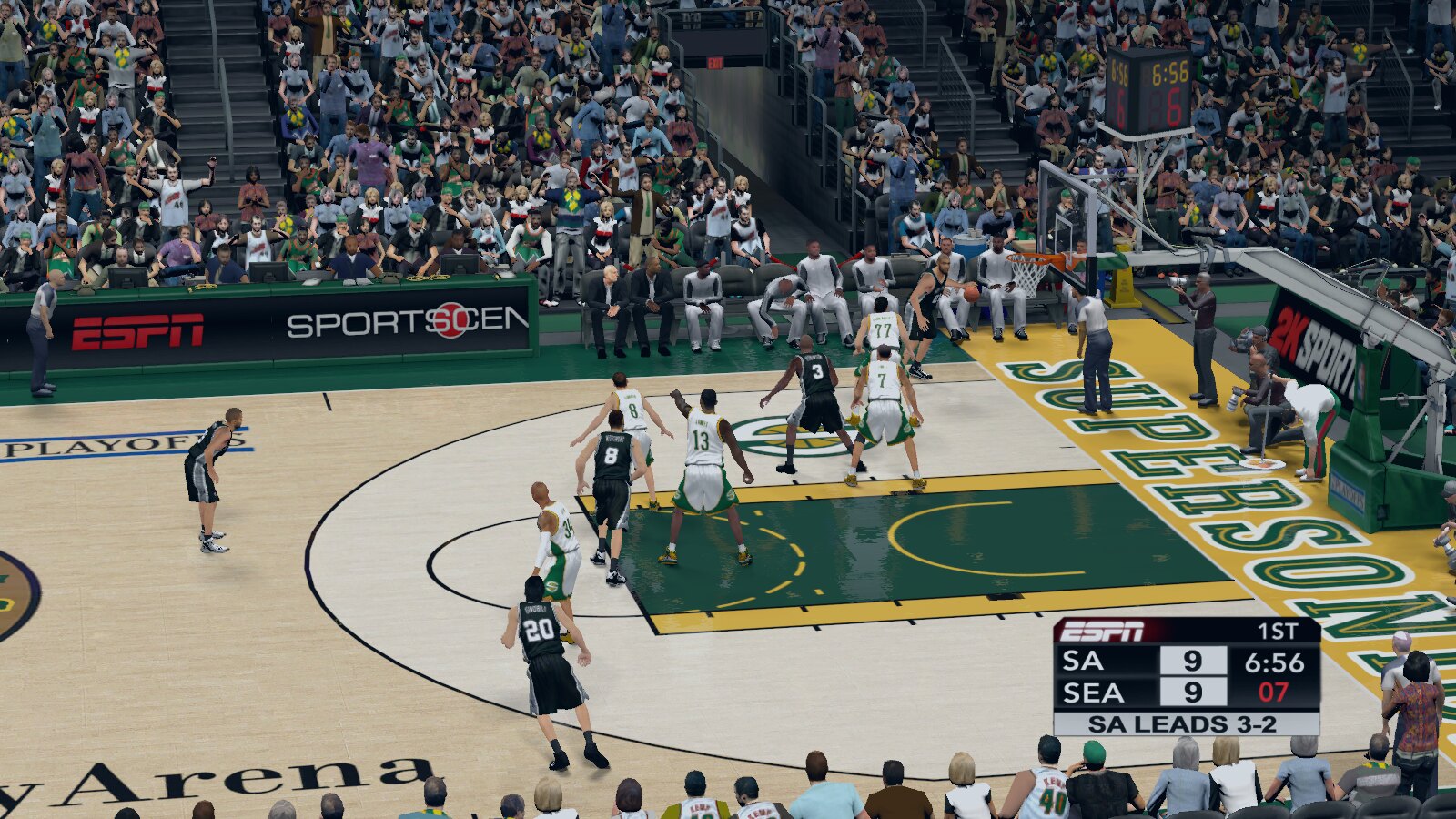This image captures an intense moment during a live basketball game. The court is adorned with vibrant green and yellow colors, prominently featuring the team name "Supersonic" on the sidelines in matching hues. In the background, spectators fill the stands, their attention riveted on the ongoing play. The court itself is bustling with activity; ten players are in the midst of the game while additional players are seated on the sidelines, awaiting their turn to join the action. 

The perimeter of the court is lined with signage from sponsors, including prominent banners for ESPN Sports Center and 2K Sports. In the bottom right corner of the image, the ESPN broadcast overlay indicates that it's the first quarter, with the game score tied at 9 points each between teams SA and CEA. It also records that SA leads the playoff series 3-2. A time clock shows that there are 6 minutes and 56 seconds remaining in the quarter, adding a sense of urgency and excitement to the scene.